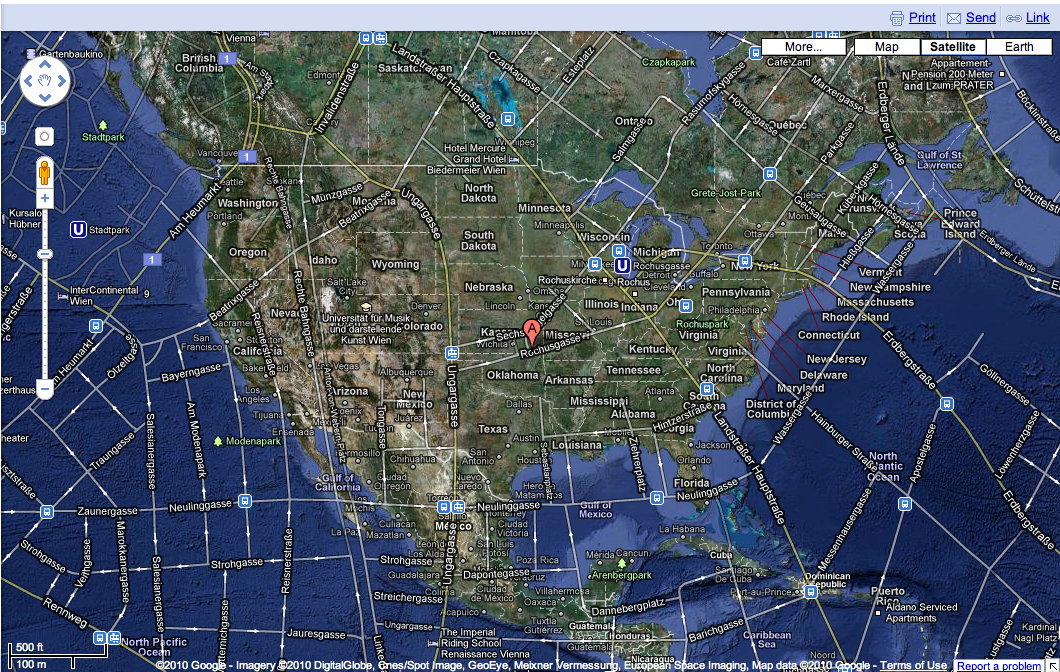This is a computer-rendered satellite image of a map, specifically a detailed screenshot of the United States of America and parts of Canada and Mexico. The terrain is depicted in shades of gray, green, and brown, indicating various elevations and landforms from rocky to flat areas. The 50 states are clearly marked with white text, each positioned on the corresponding state, and major cities are labeled as well. Surrounding the landmass are bodies of water, the oceans, shown in a gradient of light to dark blue. The left side of the image features navigation icons, including a circular pad with arrows pointing in all directions for movement, as well as zoom level indicators. In the upper right corner, there are several buttons with labels that read 'More,' 'Map,' 'Satellite,' and 'Earth.' Additionally, the bottom of the image indicates that it is sourced from Google in 2010. Overall, the map offers a comprehensive and navigable view of the United States with an array of interactive tools visible on the interface.